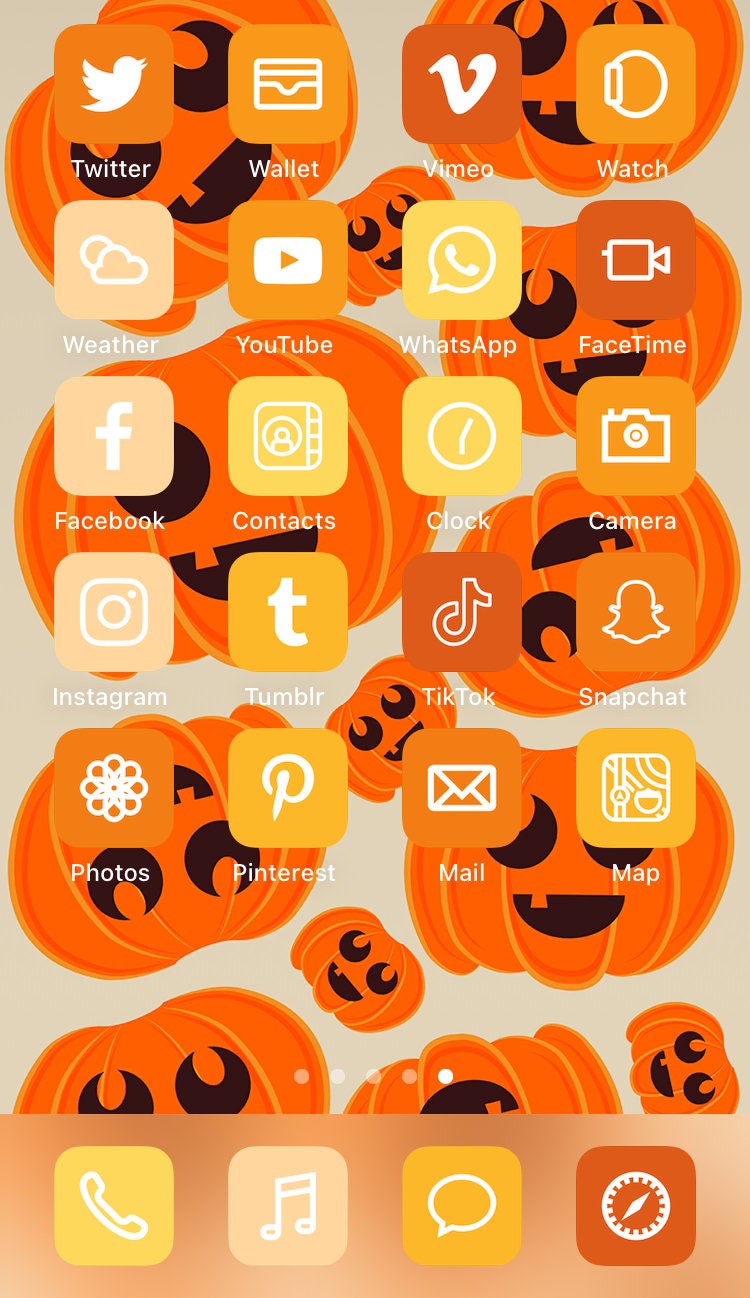A smartphone is showcased with a festive Halloween theme, featuring a colorful array of pumpkin illustrations. The pumpkins, each displaying a single-tooth grin, are scattered in various orientations—some upright, upside down, and sideways. Their cheerful faces come in autumn hues of orange, yellow, and tan. The user has an extensive collection of app icons on display, including popular ones like Twitter, Wallet, Venmo, Watch, Weather, YouTube, WhatsApp, FaceTime, Facebook, Contacts, Clock, Camera, Instagram, Tumblr, TikTok, and Snapchat. The collection also features Photos, Pinterest, Mail, and Maps. Despite the Halloween customization, the icons are predominately in muted shades of yellow, orange, and pale colors, lacking enough contrast to make them stand out vividly. At the bottom of the screen are four frequently used apps: Phone, Music, Messaging, and a peculiar version of what appears to be the Settings icon. The caption humorously notes the user's heavy reliance on social media and suggests a need to unplug. The overall festive design, although well-coordinated with the fall theme, might not appeal to everyone due to its subdued color scheme.